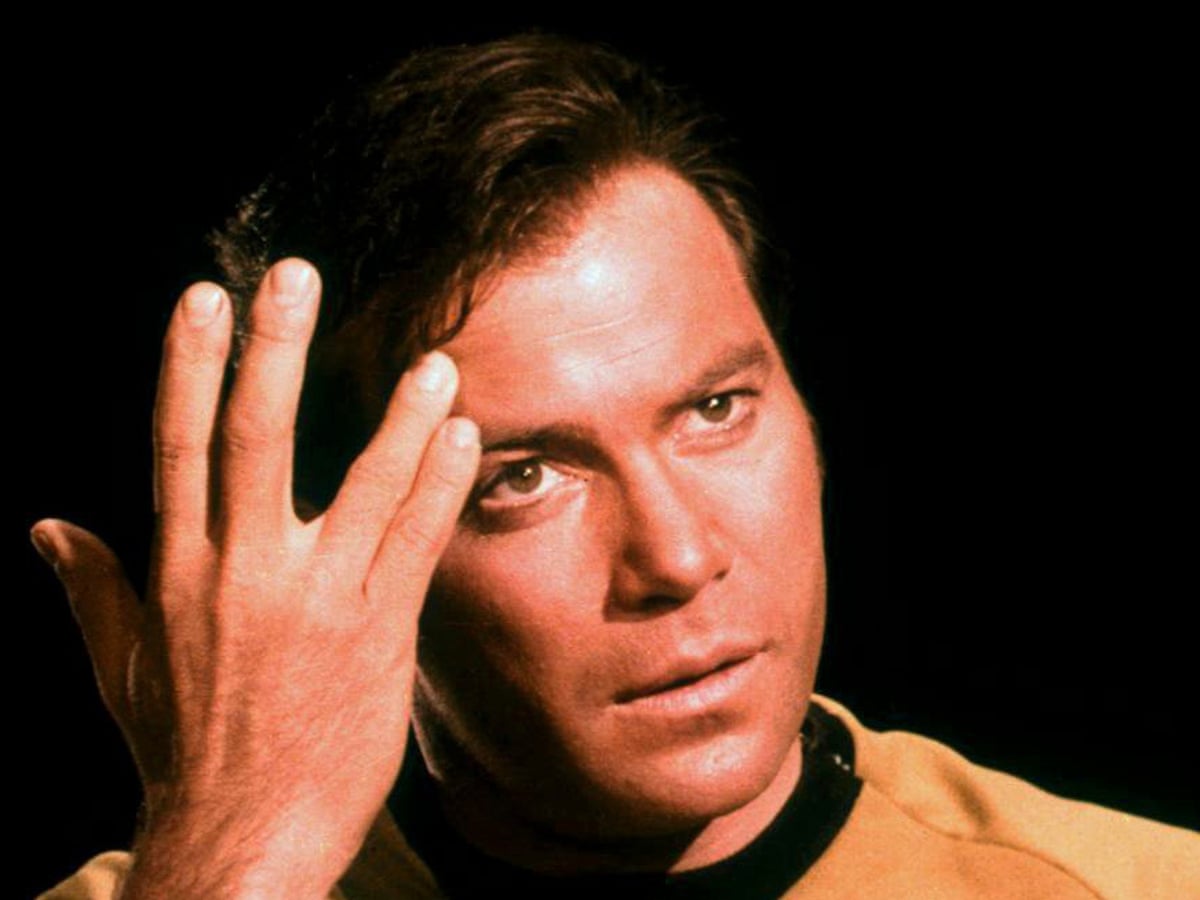The image captures a young William Shatner as Captain James T. Kirk from the 1960s TV show *Star Trek*. Shatner, dressed in his iconic gold uniform with a black collar, stands against a completely black background. His brown hair is highlighted by a light that also illuminates his face. Notably, his right hand—positioned on his forehead—forms a near "Live Long and Prosper" gesture, though the positioning is slightly off, with his ring and pinky fingers touching his forehead and his index and middle fingers extended away. Shatner gazes off to the side, not directly at the camera, his lips slightly parted, adding to the contemplative mood of the photograph.